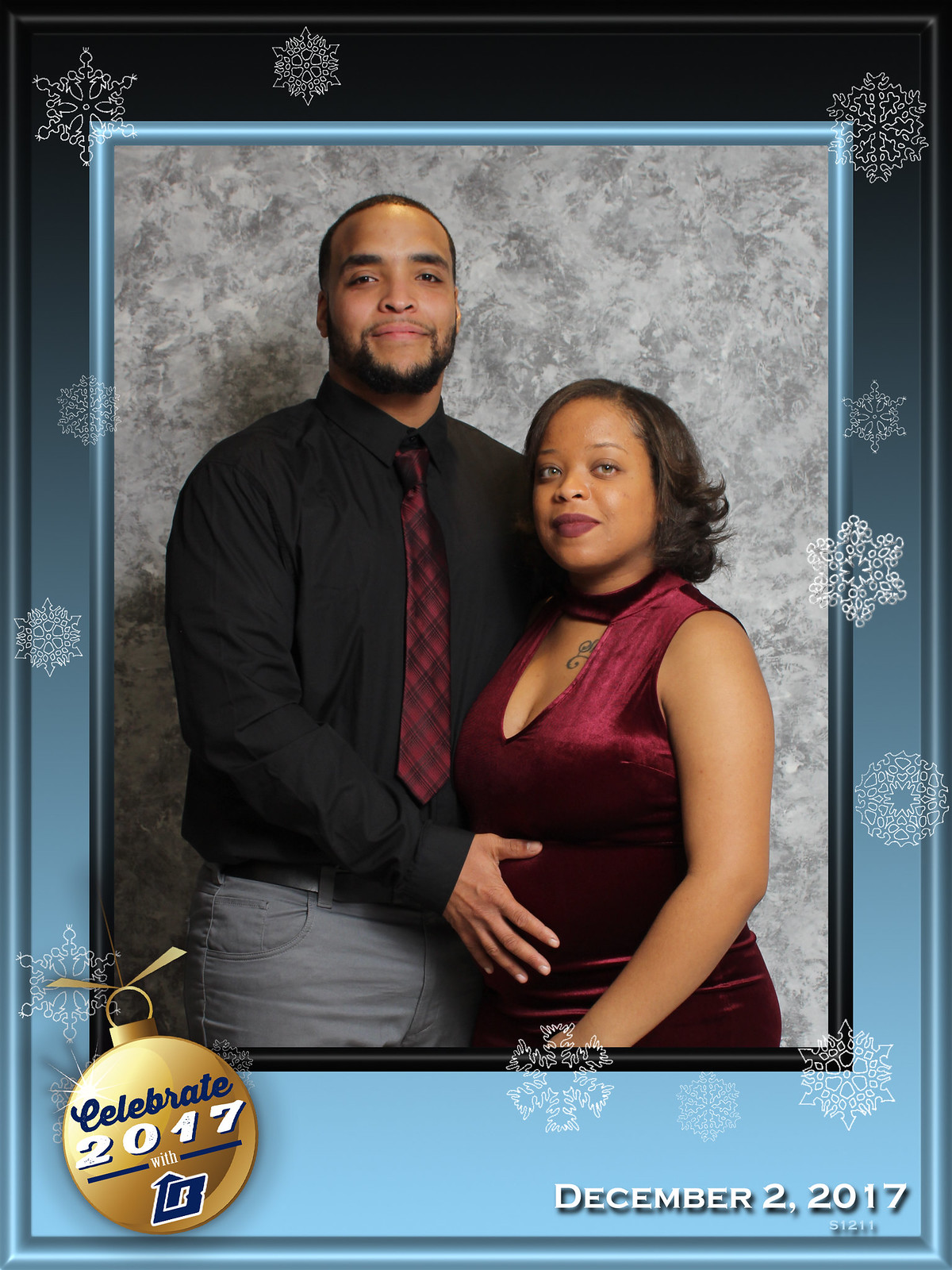This digital photograph captures a couple standing closely together and posing indoors. The man, positioned on the left, is dressed in a black button-up shirt paired with a red tie and blue jeans, with his right hand gently resting on the woman’s stomach. The woman, standing on the right, is wearing a maroon dress that reveals a tattoo on her chest. Both are smiling without showing their teeth. Behind them, the wall is a spackled grey with patterns, adding texture to the scene. The photograph is framed with a light and dark blue digital border adorned with white snowflakes, evoking a Christmas atmosphere. At the bottom left of the frame, it reads "Celebrate 2017" inside a circle, and on the bottom right, the date "December 2, 2017" is inscribed.